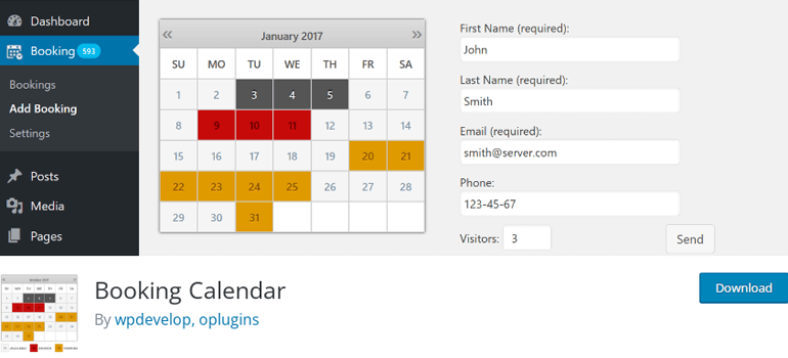The image captures a horizontal screenshot from a booking application, clearly identified as "Booking Calendar by WPDevelop" at the bottom. On the left side of the screen is a vertical, rectangular black sidebar featuring a list of menu options: Dashboard, Booking, Settings, Posts, Media, and Pages. 

Dominating the central and right portions of the image is a greyscale calendar set to January 2017. Notably, specific dates on the calendar are highlighted with varying colors: the 3rd, 4th, and 5th are shaded in dark grey; the 9th, 10th, and 11th are marked in red; and the 20th through 25th, along with the 31st, are tinted in a yellowish-orange hue.

To the immediate right of the calendar is a vertically arranged list of fields for user input: First Name, Last Name, Email, Phone, and Number of Visitors. Adjacent to these fields is a prominently placed "Send" button, followed by a blue "Download" button positioned directly beneath it.